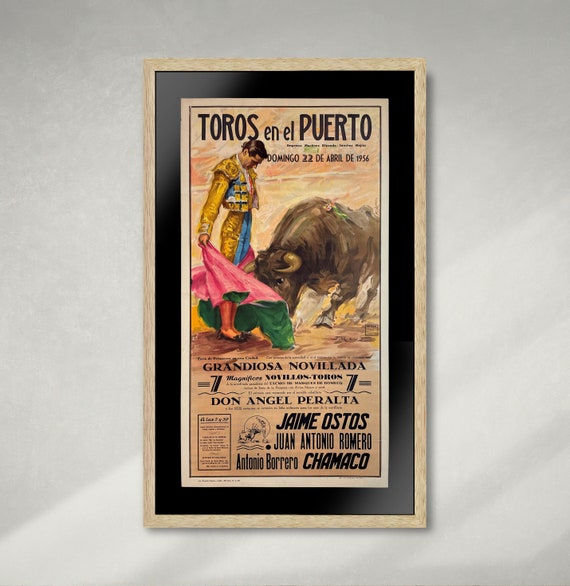Hanging against a light purple wall is a framed poster with an intricately detailed border. The frame features a beige outer rim, a black inner border, and an additional beige section inside the black border. The poster, framed within this, depicts a bullfight scene painted in a vivid animated style. Central to the image is a man dressed in a gold outfit, holding a pink cape with a green outer edge, taunting a bull to charge. The top of the poster reads "Toros en el Puerto, Domingo, 22 de Abril, D, 1956," with a grandiose description below mentioning a novella by Don Angel Peralta and featuring names like Jaime Hostos and Juan Antonio Romero in black text. The background of the poster is predominantly gray.